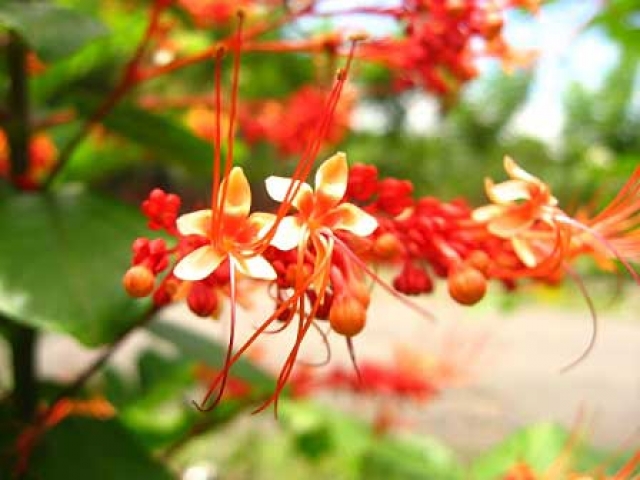This is a naturally taken, close-up photograph capturing a cluster of flowers attached to a plant. The focus reveals three open flowers with five light orange, almost cream-colored oval petals, emanating from a darker orange center. From the middle of these petals, four thin, reddish stems extend upwards, each crowned with pollen grains. Surrounding the open flowers are several unopened buds, which have a reddish and yellowish hue. Adding to the complexity, the image also shows clusters resembling red berries at the ends of red stems. The background is a blurry mix of blood green leaves and glimpses of light blue sky, providing a sense of daylight. The rich, vibrant colors of the flowers contrast sharply with the out-of-focus, green, leafy backdrop.